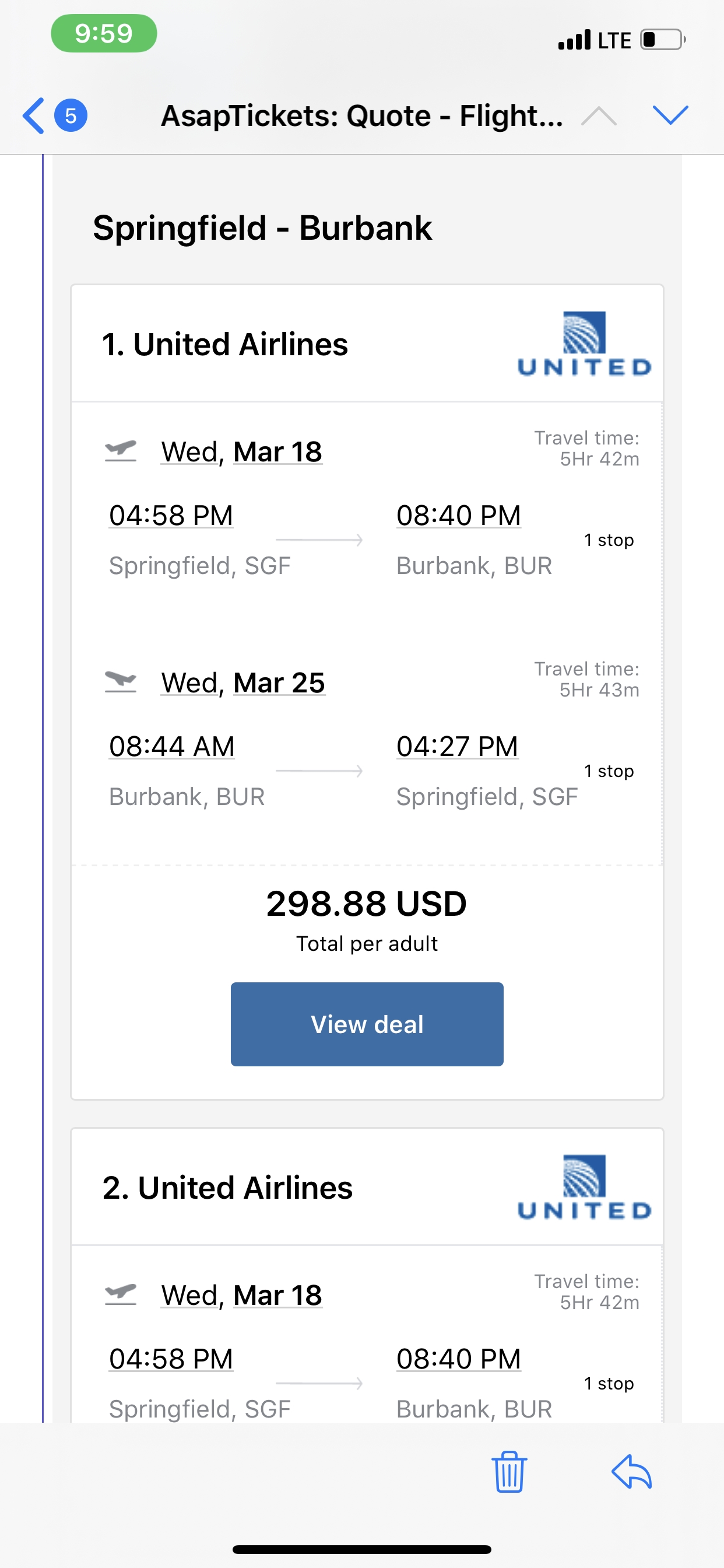A screenshot from a ticketing app, likely ASAP Tickets, displays flight quotes for a round trip between Springfield (SFG) and Burbank (BUR) with United Airlines. The outbound flight is scheduled to depart from Springfield on Wednesday, March 18th at 4:58 PM and is set to arrive in Burbank at 8:40 PM. The return flight is slated for Wednesday, March 25th, leaving Burbank at 8:44 AM and arriving back in Springfield at 4:27 PM. The total cost for this round trip is $298.88 USD per person. Another quote for an identical flight itinerary and cost appears just below, causing some confusion as there seems to be no difference between the two offers.